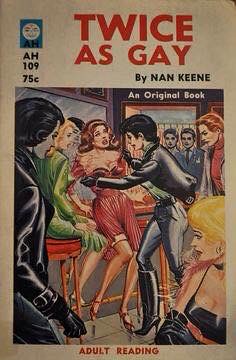The cover of the book "Twice as Gay" by Nan Keane showcases a vivid, hand-drawn illustration typical of 1950s pulp fiction style. Dominated by a scene inside a lively bar, the focus is on a woman in a red dress and red shoes, who appears startled as she is aggressively grabbed by another woman. This aggressor is dressed in a striking black leather coat, black leather pants, and knee-high, high-heeled black leather boots, with short hair suggesting a tough, biker-gang appearance. Adding to the tension, two women sit on stools next to the bar, while two men stand at the door and another lingers beside the bar. The book's title, boldly printed in red letters against a white background, is placed prominently at the top of the cover. Below it, the author's name, Nan Keane, is noted, followed by the original book label, AH 109.75, and at the bottom, it discreetly states "Adult Reading," hinting at the provocative content within.